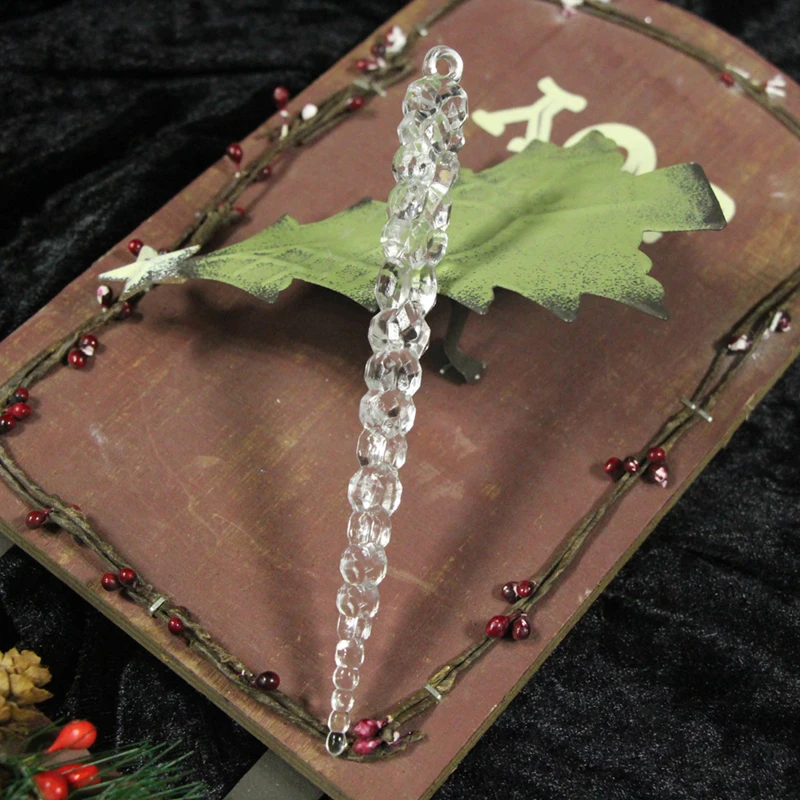The image portrays a close-up of a Christmas-themed decoration. Dominating the scene is a rectangular brown wooden plaque, set against a black crushed velvet surface. Encircling the perimeter of the plaque is decorative vinery featuring branches adorned with berries, evoking a festive atmosphere. In the center of the plaque, there is a flat, silhouetted cut-out of a Christmas tree, painted green with light distressing around the edges revealing some black. Topping the tree is a star, painted in a light yellow or white hue. 

Partially obscured by the tree cut-out, the word "Joy" is written in a white or yellowish font. Extending from one side of the plaque is a clear, braided crystal resembling an icicle, complete with a loop on top for hanging. Additional elements such as holly and small pine cones are also arranged on the black background, enhancing the holiday theme and enriching the overall festive display.